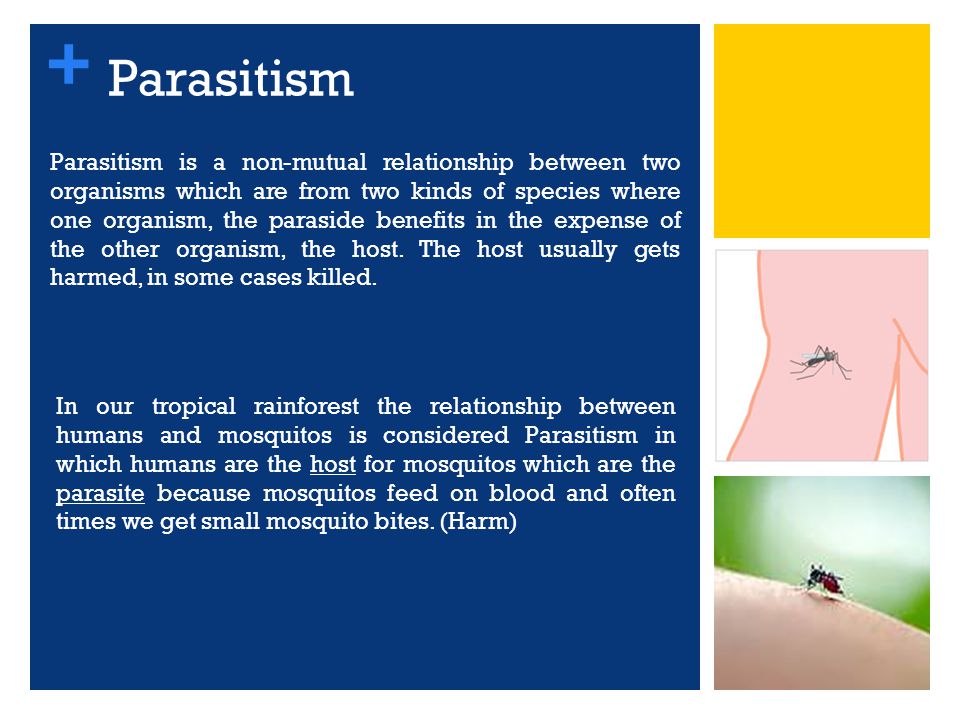The image is an informational slide on parasitism. The left side of the slide features a large blue square with white text. At the top left corner, there's a lighter blue plus sign followed by the title "Parasitism." Below it, the text reads: "Parasitism is a non-mutual relationship between two organisms, which are from two kinds of species where one organism, the parasite, benefits at the expense of the other organism, the host. The host usually gets harmed, in some cases killed." Further down, another paragraph states: "In our tropical rainforest, the relationship between humans and mosquitoes is considered parasitism, in which humans are the host and mosquitoes are the parasite because mosquitoes feed on blood and often we get small mosquito bites (harm)."

On the right side of the slide, there are three vertically aligned images the same height as the blue square. The top image is a plain yellow square. The middle image depicts a graphic representation of a mosquito poised to bite a cartooned human arm against a white background. The bottom image is a close-up photograph of an actual mosquito feeding on a real human arm, with the mosquito's body visibly engorged with blood and a green background.